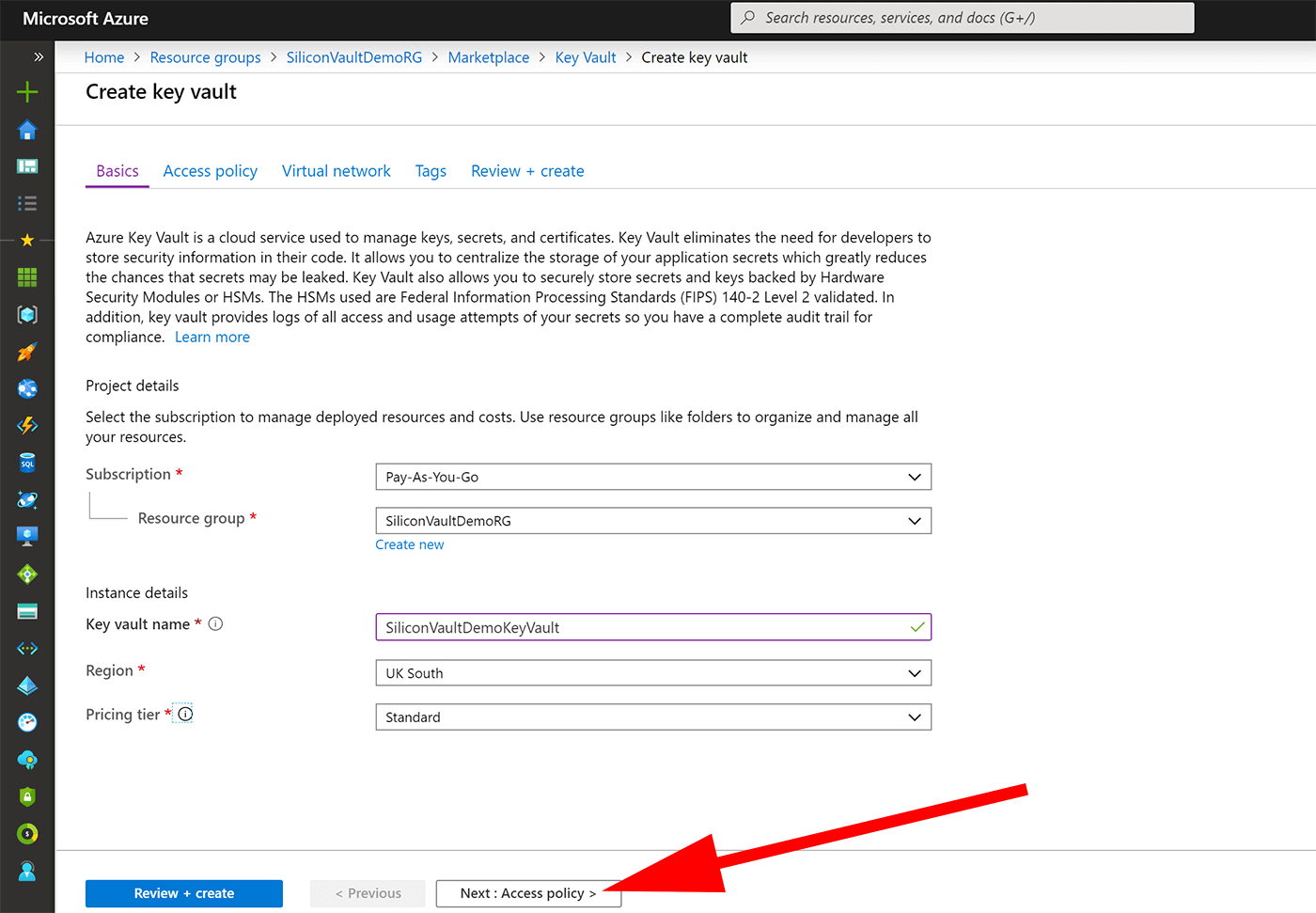The image depicts a detailed Microsoft Azure interface for creating a Key Vault. At the top of the screen, the navigation bar is visible, featuring links for "Microsoft Azure," "Home," "Resource Groups," "Silicon Vaults," "Demo," "ArcG," "Marketplace," and "Key Vaults." The user has navigated to the "Create Key Vault" page.

The interface is sectioned into different tabs: "Basics," "Access Policy," "Virtual Network," "Tags," and "Review + Create." The open tab, "Basics," provides an overview of what Azure Key Vault offers. 

Key Vault is described as a cloud service utilized for managing keys, secrets, and certificates. It explains that Key Vault removes the necessity for developers to store security information within their code, allowing for a centralized source of application secrets. This significantly minimizes the risk of secret leaks. Additionally, Key Vault enables the secure storage of secrets and keys with hardware-backed security. It further assures that access logs and usage attempts of secrets are recorded, offering a comprehensive audit trail for compliance.

Towards the bottom of the page, under "Project Details," instructions are displayed for selecting a subscription to manage deployed resources and costs. A subscription sign-up option is visible, indicating where users can enroll for the service.

Overall, the image provides a thorough instructional interface for creating and managing an Azure Key Vault, emphasizing the importance of security and compliance in protecting application secrets.